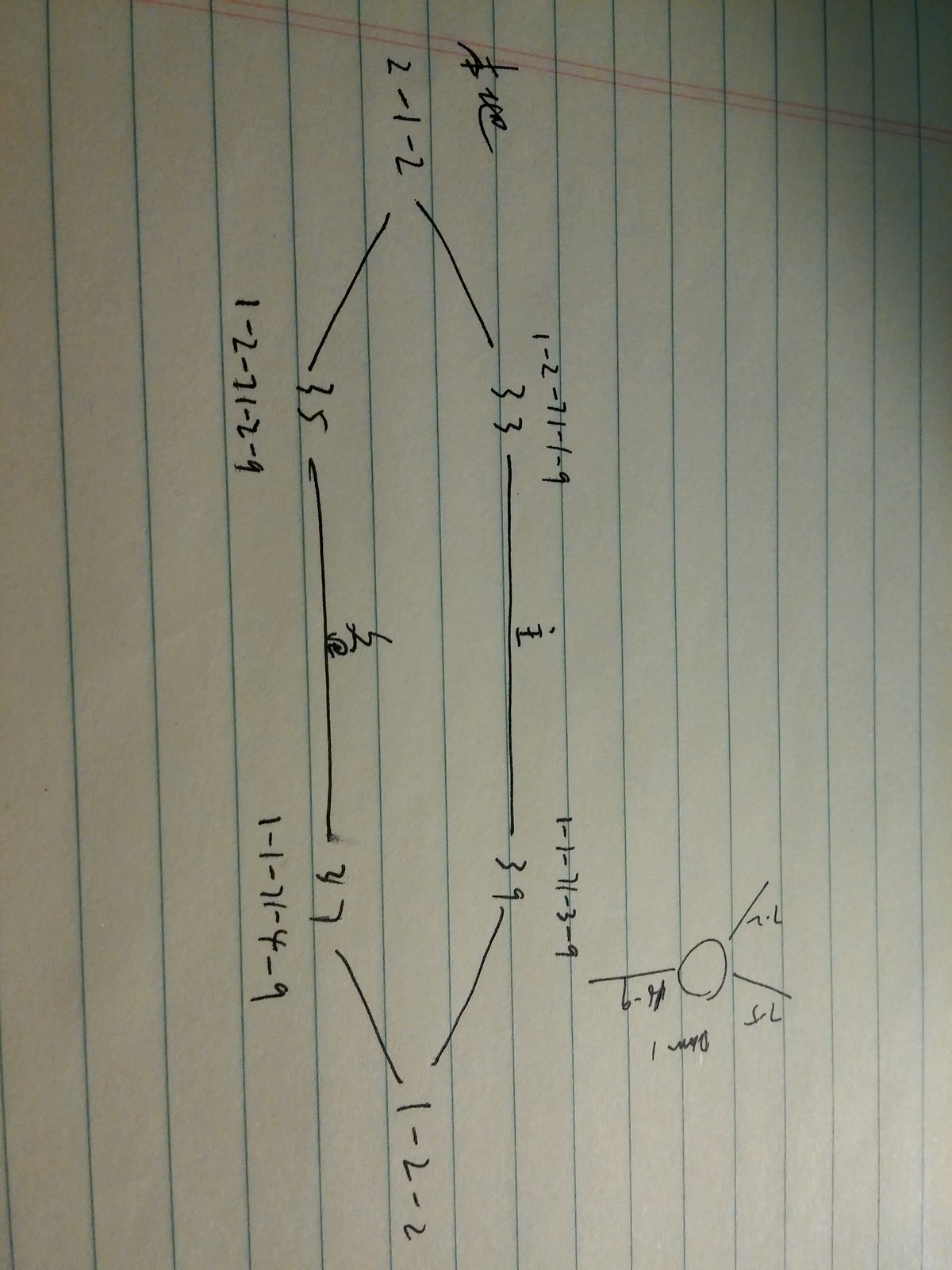This close-up image captures a single sheet of notebook paper, oriented horizontally with its blue lines running vertically. The white paper features two distinct red margin lines in the upper right corner of the visible portion. The image showcases an intricate diagram drawn in black ink, consisting of various geometric shapes annotated with multiple measurements. The annotated numbers include sequences such as 33, 1-2-2, 47, 1-1-11-4-9, 35, 1-2-7-1-2-9, and 2-1-2. At the top of one of the shapes, there is a label reading 33, followed by 1-2-71-1-9. Centrally located within the diagram is a symbol resembling a lowercase 'i' with a horizontal dash intersecting it. Every detail on the sheet contributes to a technical and precise appearance, emphasizing the meticulous nature of the diagram.